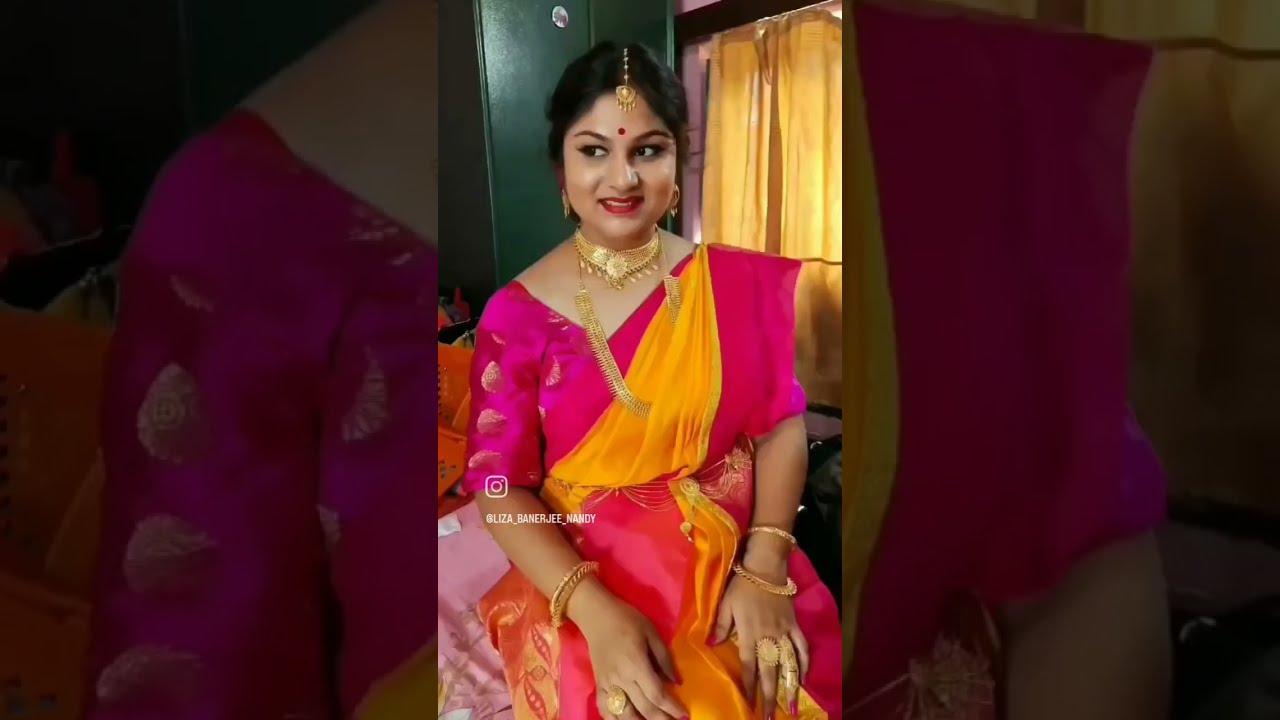This detailed photograph captures a young Indian woman seated and facing the camera. She has striking dark black hair, parted down the center, with a gold medallion on her forehead and a traditional red bindi between her eyebrows. Her makeup includes dark red lipstick, eye shadow, and eyeliner. She wears an opulent pink sari that has a shiny finish, adorned with an orangish-yellow sash that drapes stylishly across her shoulder and down the pink lower portion of her dress. Her attire is complemented by an array of jewelry: a substantial triangular-shaped gold necklace hugging her neck, alongside another longer necklace, several gold rings, and two gold bracelets on each wrist. The woman's hands rest gracefully on her legs. The background features green walls and gold curtains, and the image also includes a darkened and enlarged version of her upper torso on either side. The Instagram logo and the username "Guzza_Bonnergy_Mandy" are visible on the image. Her pose and the curvature of her body convey a sense of poised elegance, with her eyes gazing thoughtfully to her right, our left.